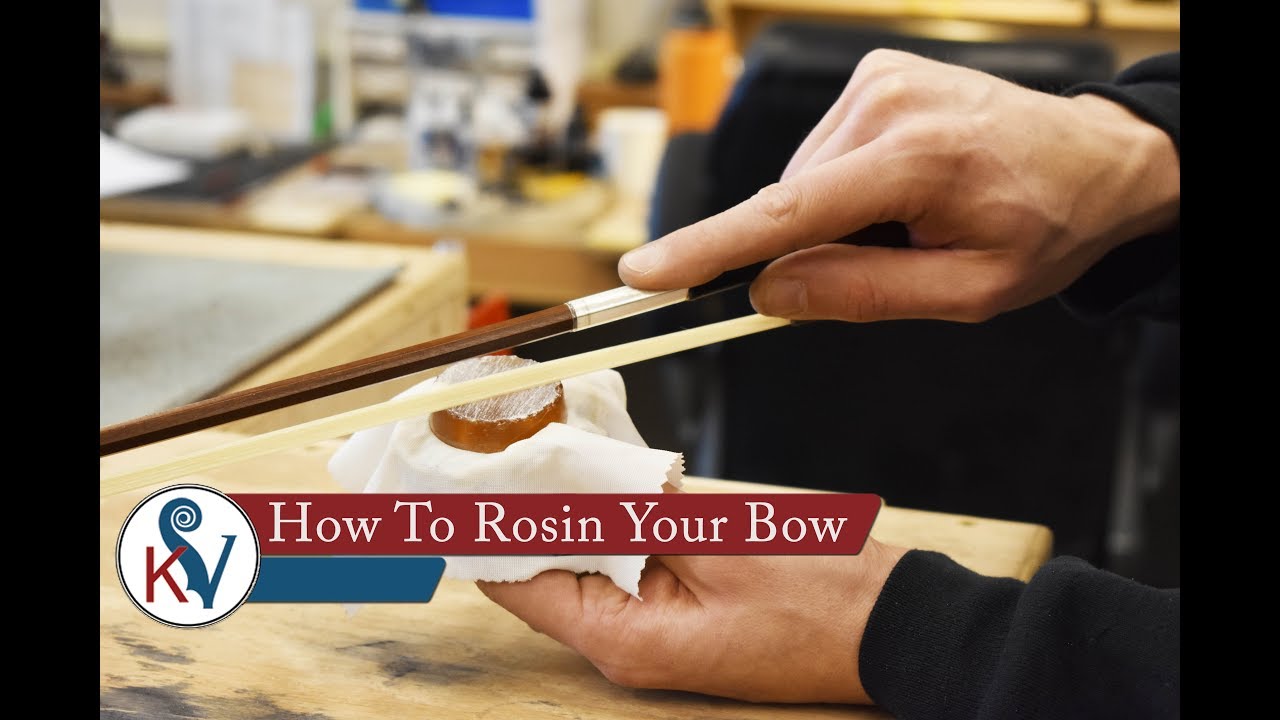A close-up image illustrates the process of rosining a violin bow. The scene features a person's hands, likely of a Caucasian individual due to the light skin tone, wearing a black sweatshirt. They are seated in front of a work area that includes a black desk chair and a wooden table with various blurred items including a cup and a mug. The person holds a piece of rosin wrapped in a white cloth with their left hand, while their right hand methodically drags the bow across it. The bow, painted with white on one side and brown on the other, also has tape in its middle. In the background, there's a subtle light from a ceiling fixture. A maroon ribbon at the bottom of the image reads "How to Rosin Your Bow" in white Garamond font. Additionally, a white circle on the left side has the letters 'K' in red and 'V' in blue, with the 'V' featuring an end resembling a violin scroll.